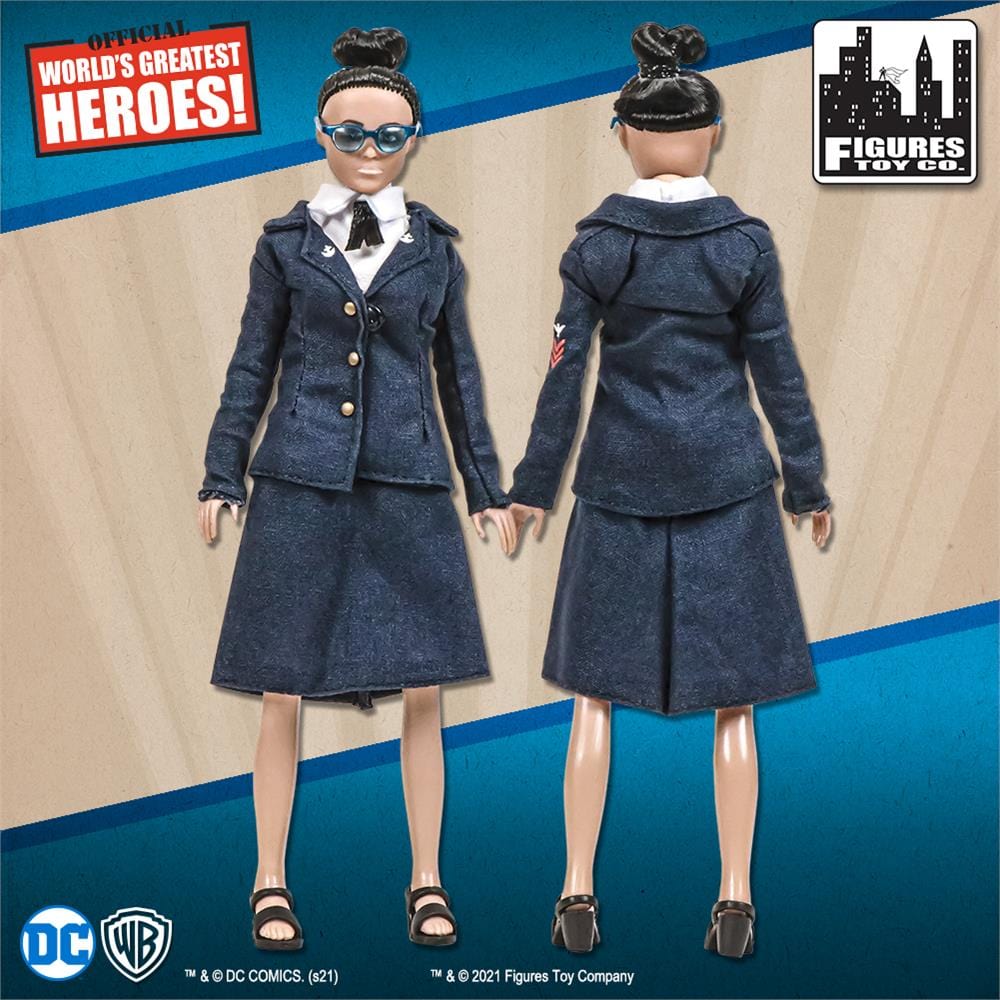This image depicts a collectible doll from Figures Toy Company, showcasing both the front and back views of the figure. The doll features black hair styled in a bun and is accessorized with blue-framed goggles. She wears a white shirt with a black ribbon-tie, and a coordinated denim jacket with three gold buttons along with a knee-length, flared denim skirt. The outfit is complemented by black heel sandals. Notably, the left sleeve of the jacket displays a logo with three V-shapes and an eagle, possibly an army insignia.

Text elements surround the doll, enhancing the advertisement's details. In the upper left corner, within a red square, the phrase "Official World's Greatest Heroes" is written in white letters. The upper right corner contains a graphic of a city's silhouette with the text "Figures Toy Company" beneath it. At the bottom of the image, there's a blue circle containing the DC and Warner Brothers symbols, along with small text reading "© DC Comics S21 TM & © 2021 Figures Toy Company."